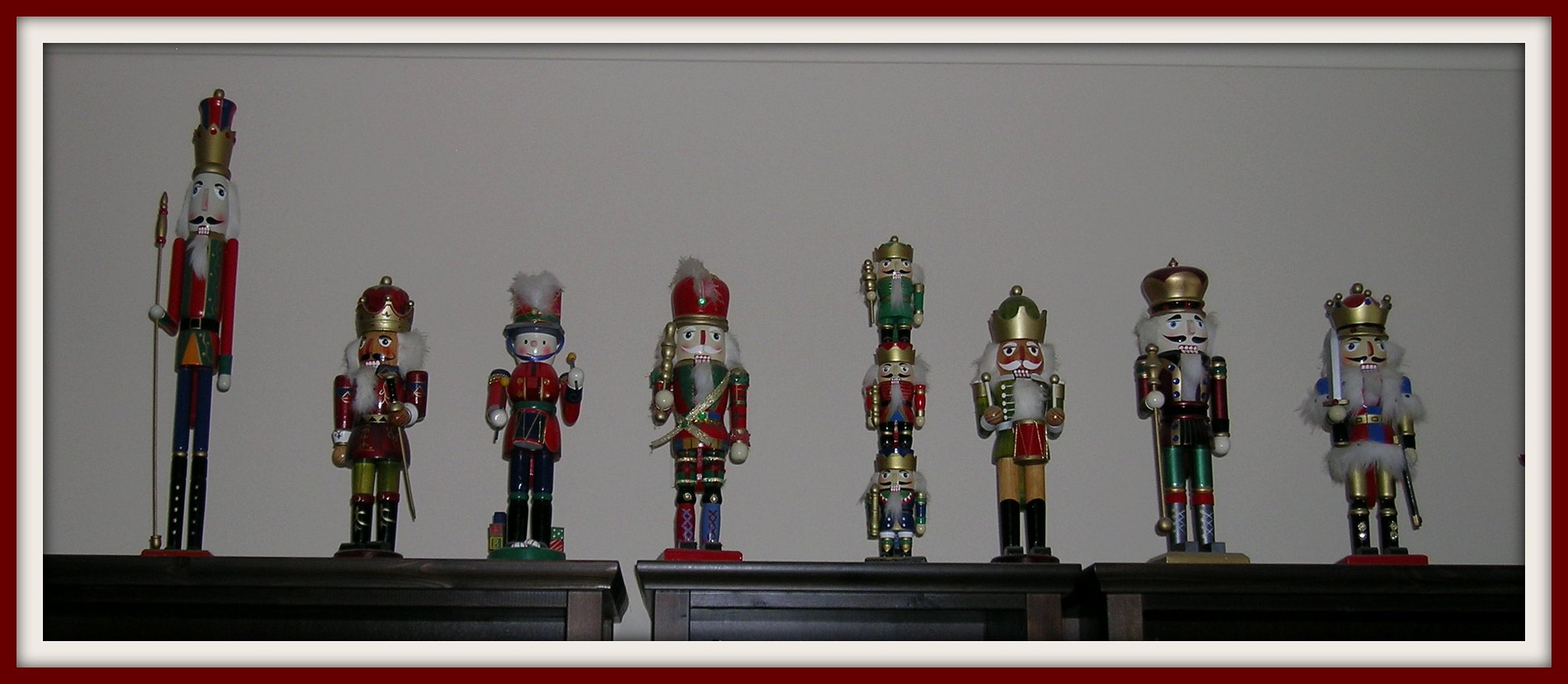This photograph, framed in a red and white border, showcases an impressive collection of eight intricately designed nutcrackers arranged in a lineup on a dark brown surface, possibly a shelf or table, against a white background. The tallest nutcracker, adorned with a mustache, long white hair, and a dual-colored crown (gold and blue-red), stands on the far left holding a spear. Beside it is a much shorter nutcracker with a king's crown and a sword but no mustache. The third figure departs from the traditional nutcracker aesthetic, resembling a snowman with a top hat and a snare drum. Next, there's another white-haired, mustached nutcracker carrying a small stick. In the center, three small nutcrackers stacked on top of each other, colored green, red, and blue, add a playful touch to the display. To their right is a nutcracker with white hair and a green crown, followed by a black-mustached, white-haired nutcracker. Finally, the last figure, bearing a king's crown, white mustache, and sword, completes this charming and diverse nutcracker assortment.